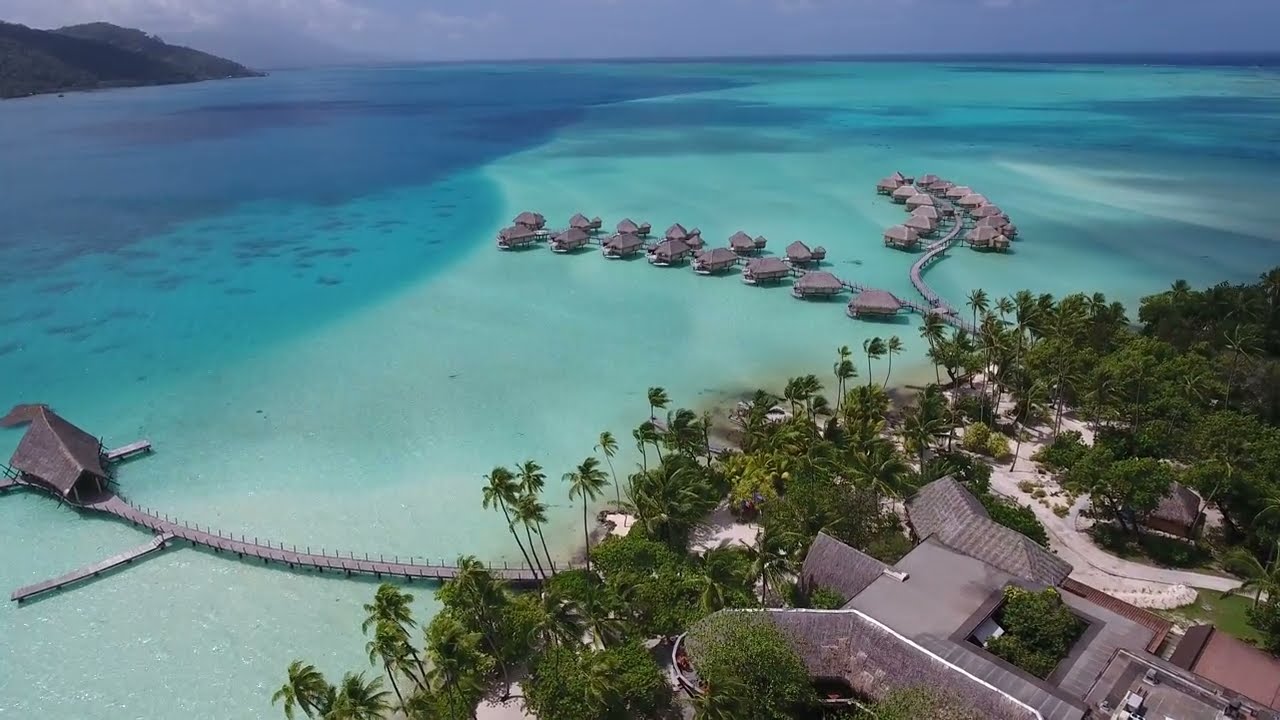This aerial photograph captures a vibrant, sunlit scene featuring a cluster of tall, green palm trees with their characteristic long, thin leaves. These palms line a small, glistening pond, partially obscured by the dense foliage. The bright green grass and lush weeds contrast with a sandy dirt area located to the right of the trees. Surrounding the pond on the left is a jungle-like assemblage of various green plants, shorter trees, and dense foliage, all bathing in the brilliant sunlight. The reflection of the palm branches can be seen on the water's surface, merging with glimpses of the pond's bottom. No sky is visible in the frame, focusing all attention on the greenery and the serene body of water below.